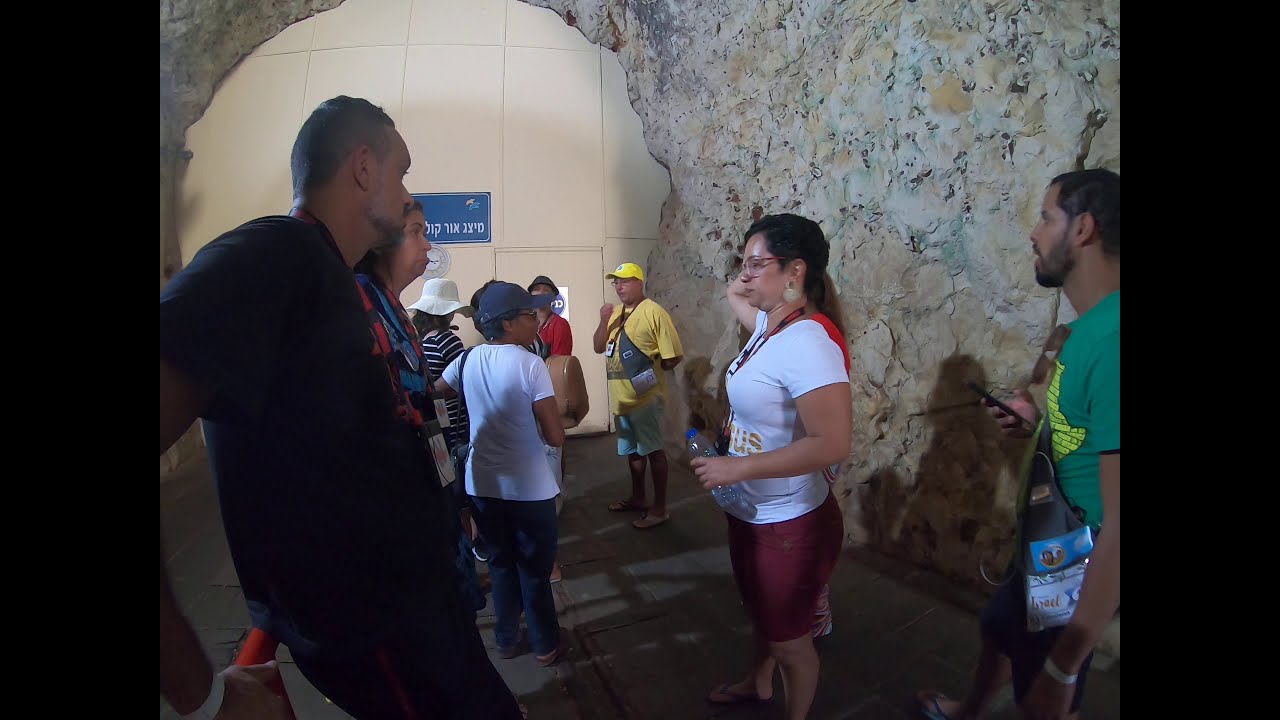The image displays a group of people standing in an informal, somewhat disorganized line, facing mostly in the same direction. They seem to be indoors, possibly in a location with a cave-like aesthetic. The scene is bounded by a rough, light gray rock wall with tan patches on the right, and a red metal railing on the left side of the walkway. The people are in leisure attire, with many wearing t-shirts and shorts. A prominent figure is a man wearing a green shirt with an unreadable, light green text, holding a blue pamphlet. Beside him is a woman in a white shirt and red pants, holding a water bottle. In the background stands a possible tour guide, dressed in a yellow shirt, yellow hat, and light blue pants, speaking into a microphone. Among the crowd are individuals who seem to be of Asian descent, with one woman in a red shirt wearing a black face mask. Another notable person is a woman in a white hat with a black-and-white striped shirt. The group is gathered near the end of the walkway, which leads to a large tiled wall with a blue sign featuring white Asian characters. This mix of observations paints a vivid picture of a diverse group of people waiting in line in a rocky, cave-like passage.